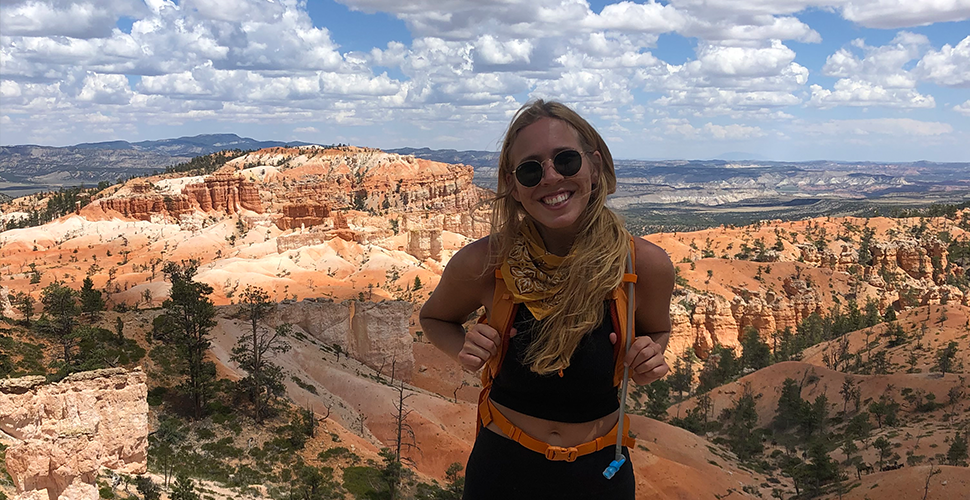In this photograph, a young Caucasian woman with long blonde hair stands at the center, her locks cascading down to her chest. She dons circular black sunglasses and is smiling brightly, revealing her white teeth. Her sleeveless black top exposes her midriff, complemented by a distinctive orange belt. She's clad in black pants and holds an orange backpack equipped with a water pipe draped over her front. An array of colorful pins adorns her outfit, along with a yellow neck scarf. Behind her stretches a breathtaking landscape featuring puffy white clouds in a light blue sky, characteristic evergreen trees, and expansive rocky formations suggestive of a desert or mountainous region, with a mix of green and brown patches. This image, possibly taken during a hike, captures the serene beauty of the natural surroundings and the woman's vibrant and adventurous spirit.